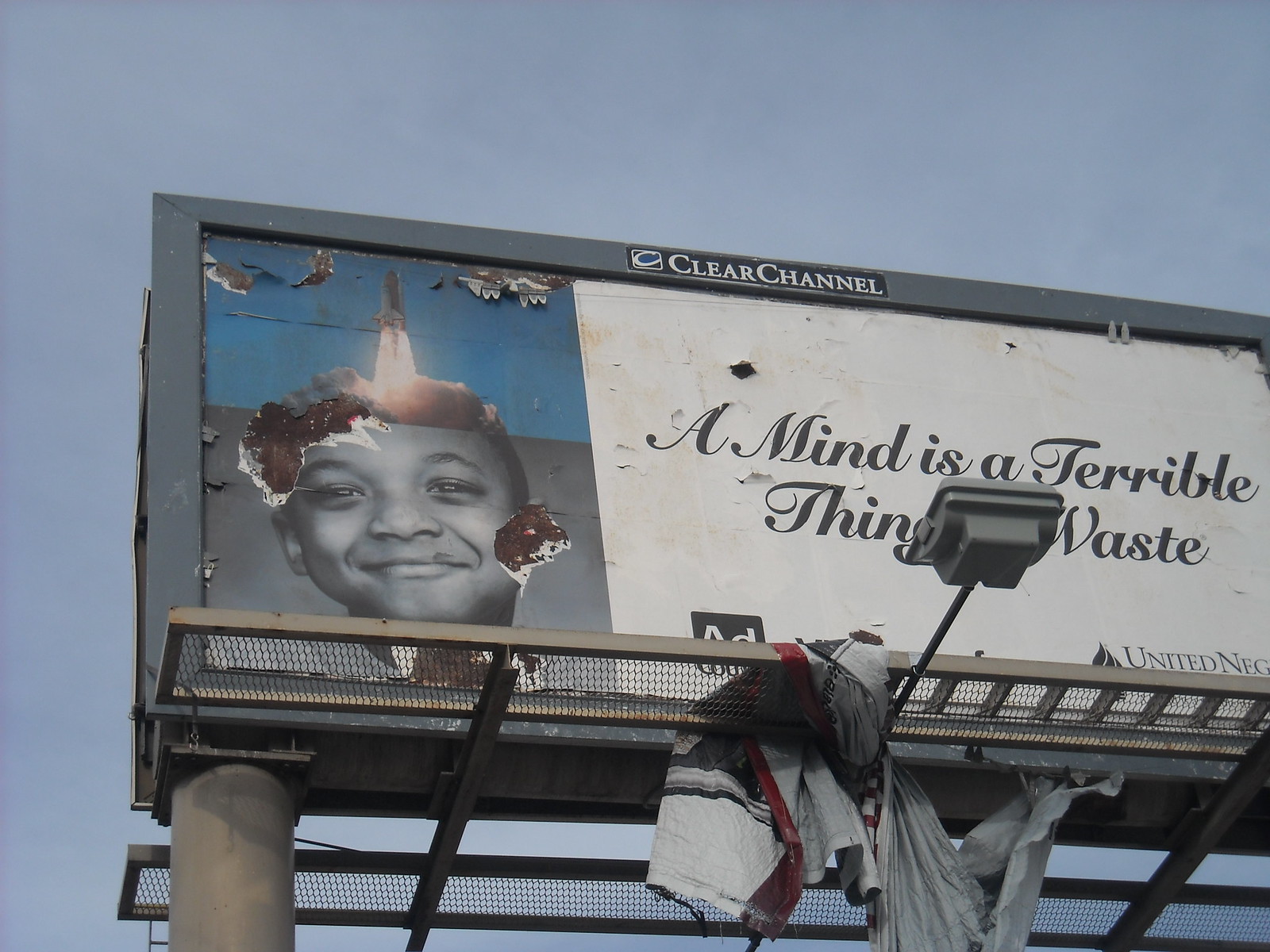The image captures a weathered billboard under a clear blue sky. The billboard's metal frame and grated walkway, designed for maintenance work, show signs of deterioration, with peeling paint and torn paper scattered across its surface. A nearly illegible Clear Channel Communications logo perches at the top, signaling the ownership.  

On the left-hand side of the billboard, a partially damaged black-and-white photograph of an African American boy is visible, though parts of his head and cheek are missing due to the peeling layers. Above this image, a vibrant blue background depicts a space shuttle blasting off into space. To the right of the boy's face, the message "A Mind is a Terrible Thing to Waste" is written in cursive black text against a white backdrop. Logos for the Ad Council and the United Negro College Fund are positioned beneath this phrase. 

Additional damage is evident as sections of the poster hang loosely from the metal grating, indicating a state of neglect. Moreover, a tattered gray-striped t-shirt is tangled in the walkway’s structure. The billboard stands atop a cement pylon, struggling to maintain composure against the elements, contributing to the overall sense of decay.